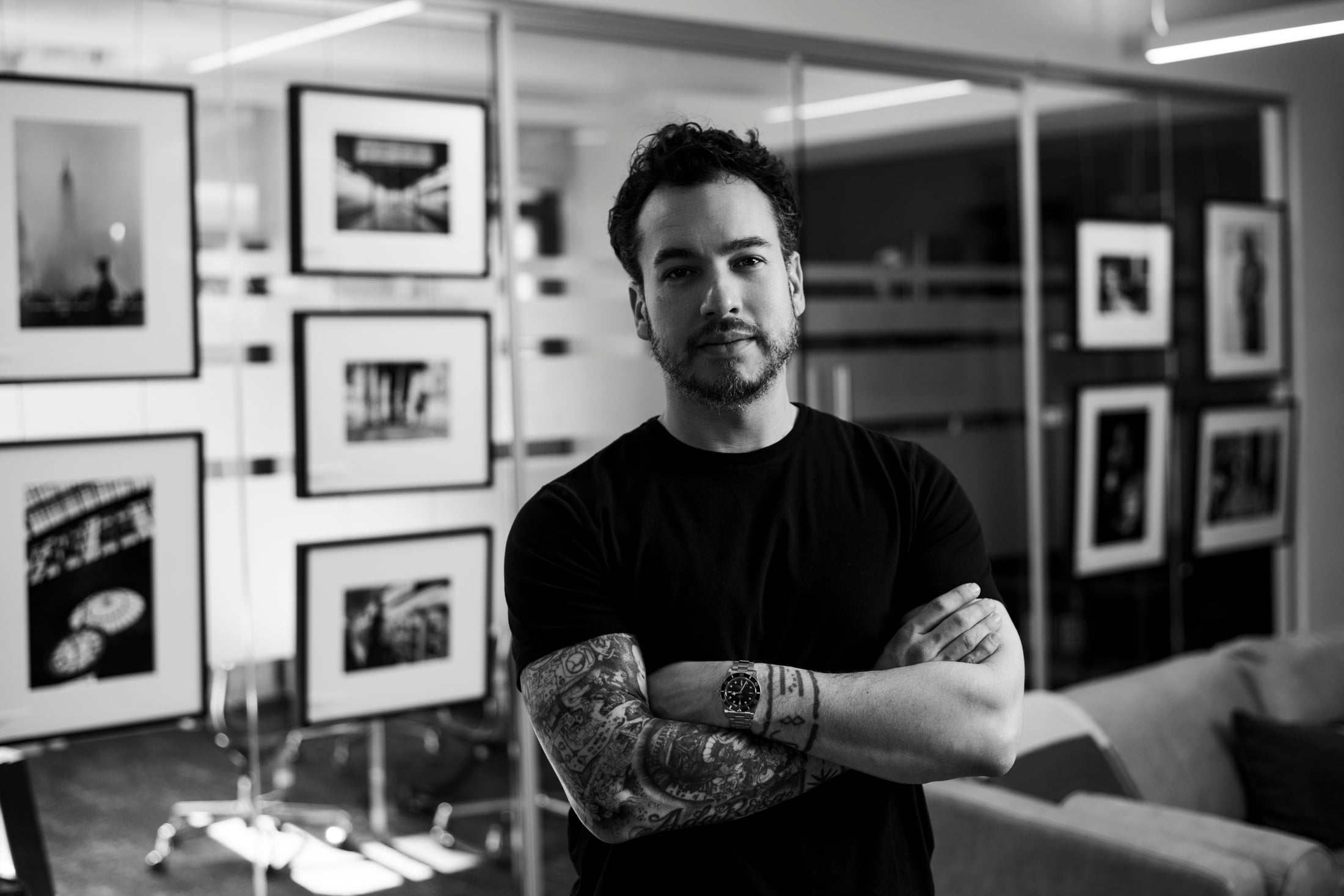The image features a man in his early 30s, standing with his arms crossed at the center to center-right of the composition. He has dark, wavy hair, a short beard, and a mustache, with a hint of gray. His thick black eyebrows and black eyes give a direct stare into the camera. He is dressed in a black short-sleeved t-shirt, showcasing tattoos: a full sleeve tattoo on his right arm and a smaller, wrist tattoo on the left, just below a silver watch with a black face. The image is entirely in black and white. To his right, there's a gray sofa adorned with black cushions. The backdrop consists of a glass wall adorned with framed pictures, some depicting famous landmarks like the Eiffel Tower and buildings. Through the glass wall, one can glimpse additional spaces, including possible chairs to the left and shelves to the right, suggesting a complex background that adds depth to the image.